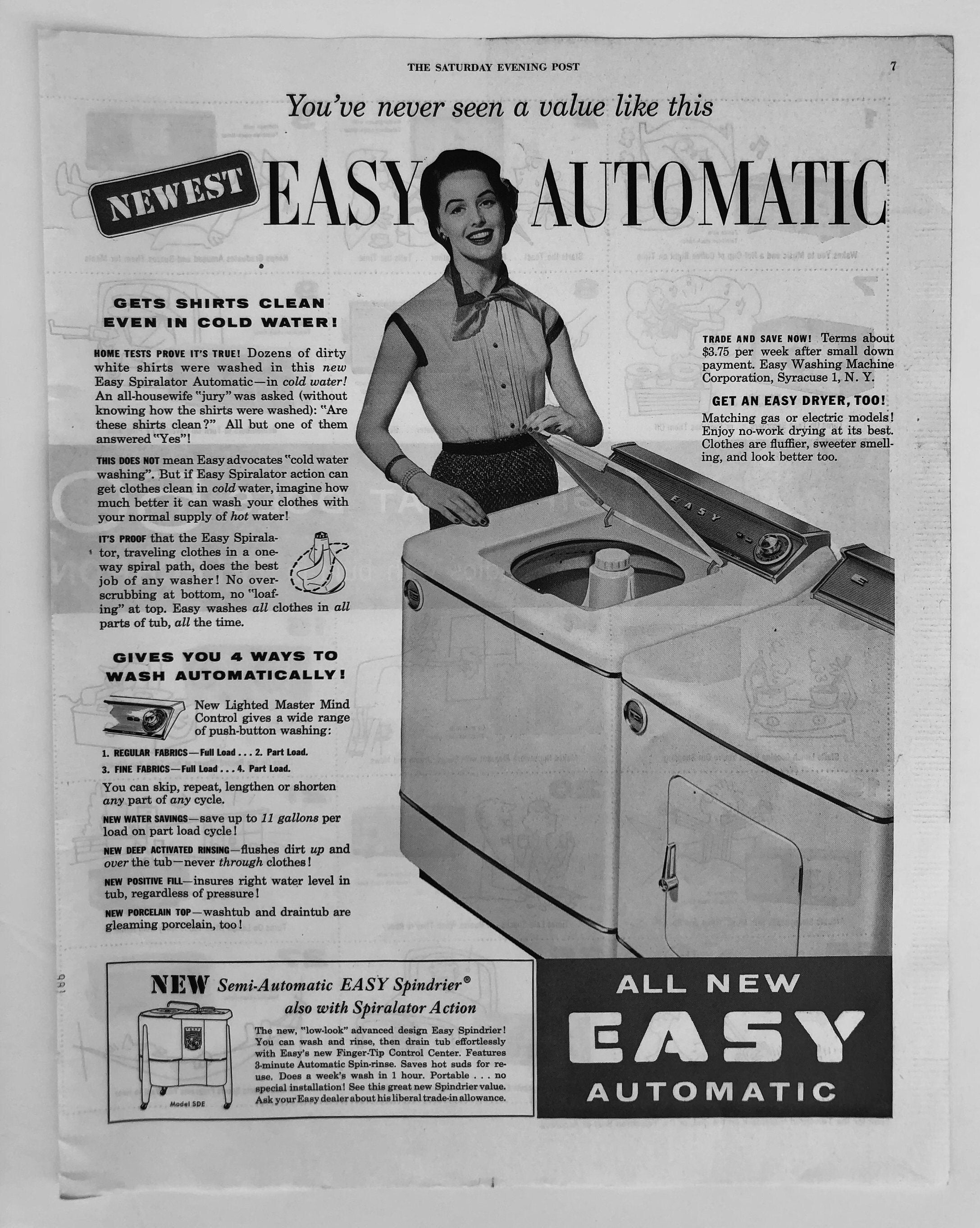This black-and-white advertisement is likely from the 1940s or 1950s and appeared on page seven of the Saturday Evening Post. It features a neatly dressed woman wearing a short-sleeve button-down shirt, a skirt, and a scarf around her neck, styled in 1950s fashion with short, wavy hair and bright lipstick. Smiling, she stands beside a washing machine, lifting its lid to reveal the agitator inside. The brand "EZ" is prominently displayed on the control panel. Beside the washing machine is a matching dryer unit. The headline reads, "You've never seen a value like this. Newest EZ Automatic." The ad includes multiple paragraphs extolling the features and benefits of the washing machine, highlighting its ability to get shirts clean even in cold water. Additionally, the ad promotes the new semi-automatic EZ spin dryer with spiralator action. The backdrop of the page is a light gray, further emphasizing the contrast of the black-and-white print.